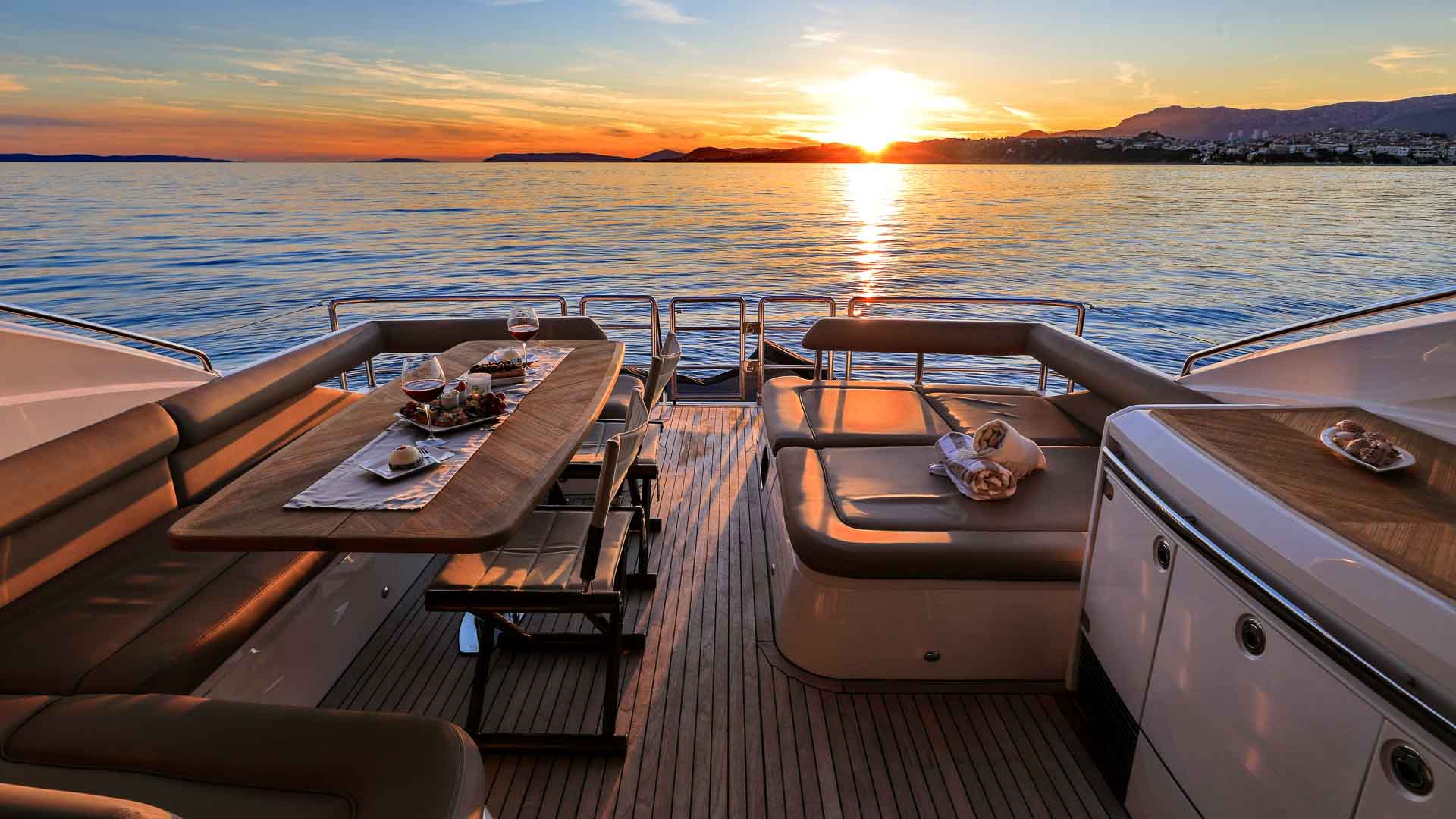The full-color landscape photograph captures an idyllic scene aboard a luxurious yacht at sea, framed horizontally with natural light just moments before sunset. The yacht's back deck, featuring a wooden floor and white interior, overlooks calm, dark blue waters. The upper portion of the image reveals a sky adorned with beautiful clouds painted in glowing red and orange hues by the near-setting sun, perched just above the horizon. In the background, a coastline dotted with buildings and distant hills is visible, adding depth to the tranquil setting.

On the deck, a tastefully staged dining area is set on the left, complete with a wooden table draped in a white tablecloth. The table features a centerpiece runner adorned with glasses of red wine, assorted desserts including cakes and cheese, and possibly other food items. Wooden chairs and a cushioned booth are arranged around the table, inviting relaxation and comfort. To the right, a spacious mattress with folded blankets promises a restful lounging spot, ensuring all elements of luxury and leisure are captured in this serene, people-free moment aboard the yacht.